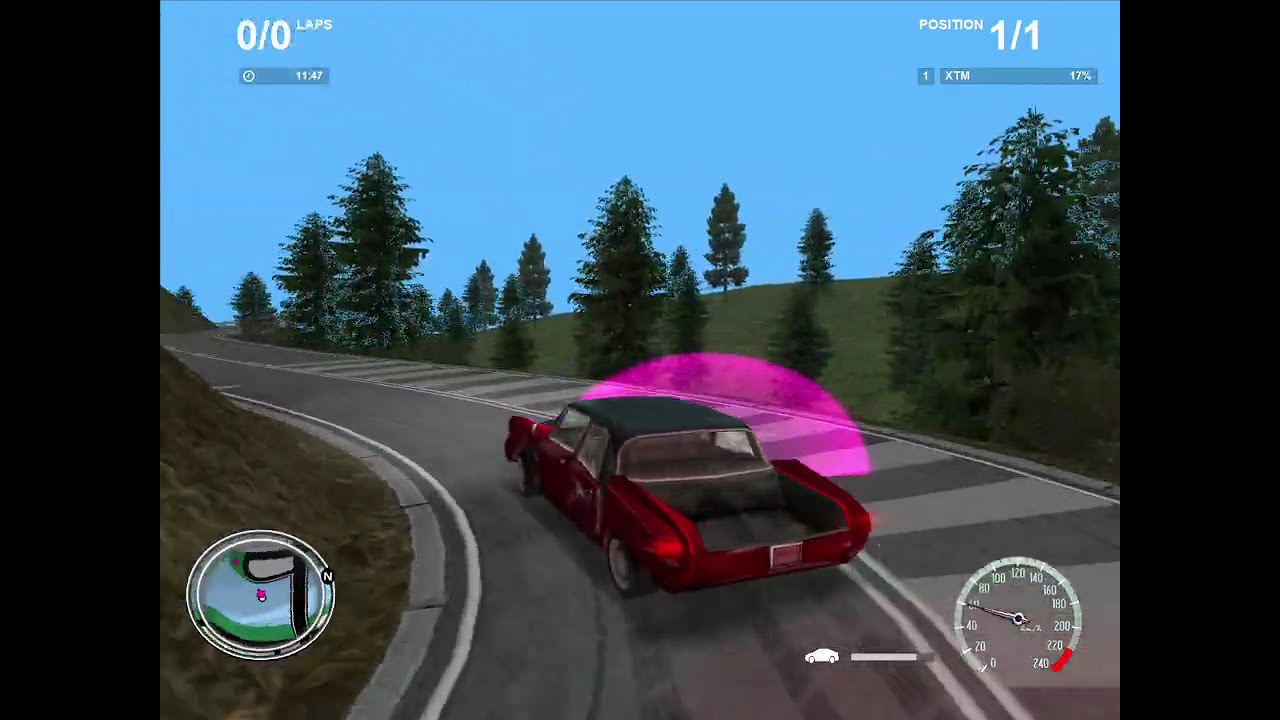The screenshot, depicting a racing video game reminiscent of Nintendo 64 graphics, showcases a vibrant scene with a red sports car navigating a hilly, winding road that curves to the left. The car, with a notable pink halo above it and missing its trunk, is shown driving along a two-lane gray road marked with double white lines. On the right side, lush grass and trees contrast against the hilly terrain on the left, all under a clear blue sky. Overlaying the image is a comprehensive heads-up display: a circular race map in the bottom left corner, a speedometer in the bottom right corner indicating the car's speed, and a position marker in the upper right corner showing a status of "Position: 1/1." Additionally, the top left corner displays "0/0 Laps" along with a time reading of "11:47." The image includes white horizontal blocks on both far sides, adding to the retro game aesthetic.